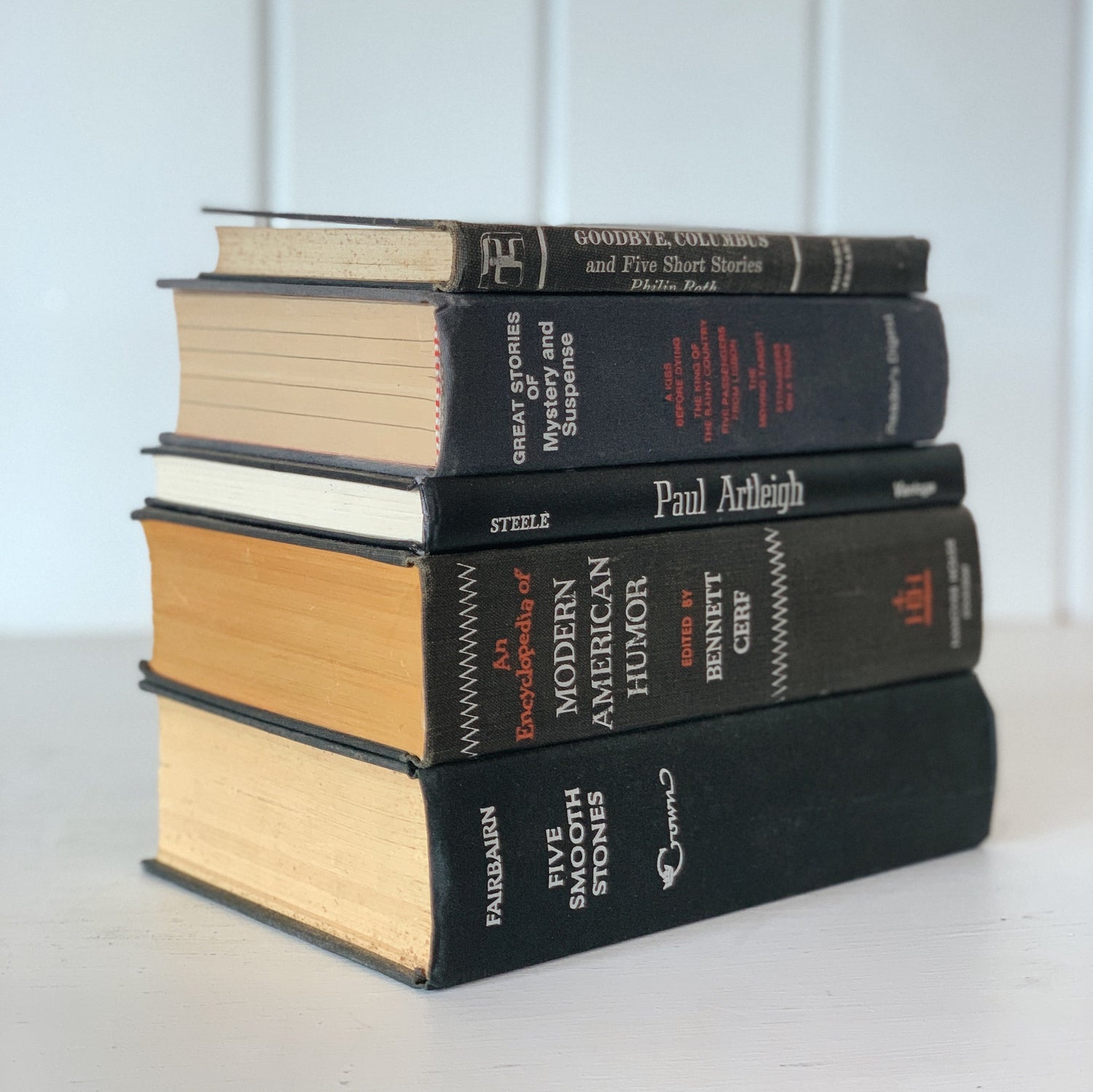The image depicts a carefully arranged stack of five books of varying thicknesses, positioned at an angle from the bottom left to the top right. The books are resting on a light gray surface, against a background featuring a white wall with vertical gray panel lines. 

From top to bottom, the titles are as follows: 

1. "Goodbye, Columbus and Five Short Stories" by Philip Roth—this book has a dark gray cover and is slightly bent open.
2. "Great Stories of Mystery and Suspense"—a book with a bold blue cover and red text below the title that's too small to read.
3. "Steel" by Paul R. DeLay—this is a thinner black book, with an additional word at the end that is out of focus.
4. "An Encyclopedia of Modern American Humor" edited by Bennett Cerf—this is a very thick black book featuring a zigzag design at the top and bottom, with red and white text.
5. "Five Smooth Stones" by Fairbairn—the book at the bottom is dark black with white text, including a cursive signature that reads "C-O-W-N." 

The photography style is representational realism, capturing the detailed texture and titles of the books while maintaining focus on the neat arrangement and stacked design.